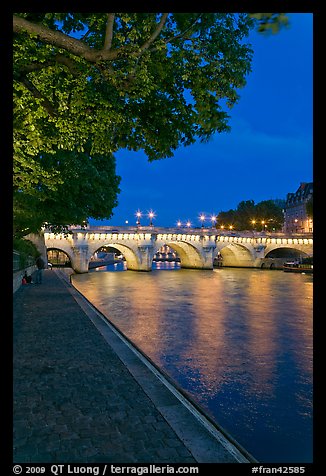This nighttime photograph depicts a beautifully lit bridge extending across a calm river. The bridge, illuminated by lights both above and below, creates a striking contrast against the clear, dark blue sky, also adorned with patches of clouds in varying shades. On the left side of the image, an old stone walkway passes beneath the bridge, accompanied by lush green trees and a prominent tree overhanging the water, occupying about half of the picture. The walkway, partially cobbled, stretches along the river bank where two figures can be discerned—one sitting and another mid-stride. The bright lights from the bridge reflect off the water in the foreground, adding to the serene ambiance. At the bottom of the image, the text "#Fran42585" is visible in white. This image, originating from TerraGalleria.com and dated 2009, captures a tranquil cityscape with no other people in sight, emphasizing the peaceful and well-lit environment perfect for an evening stroll.